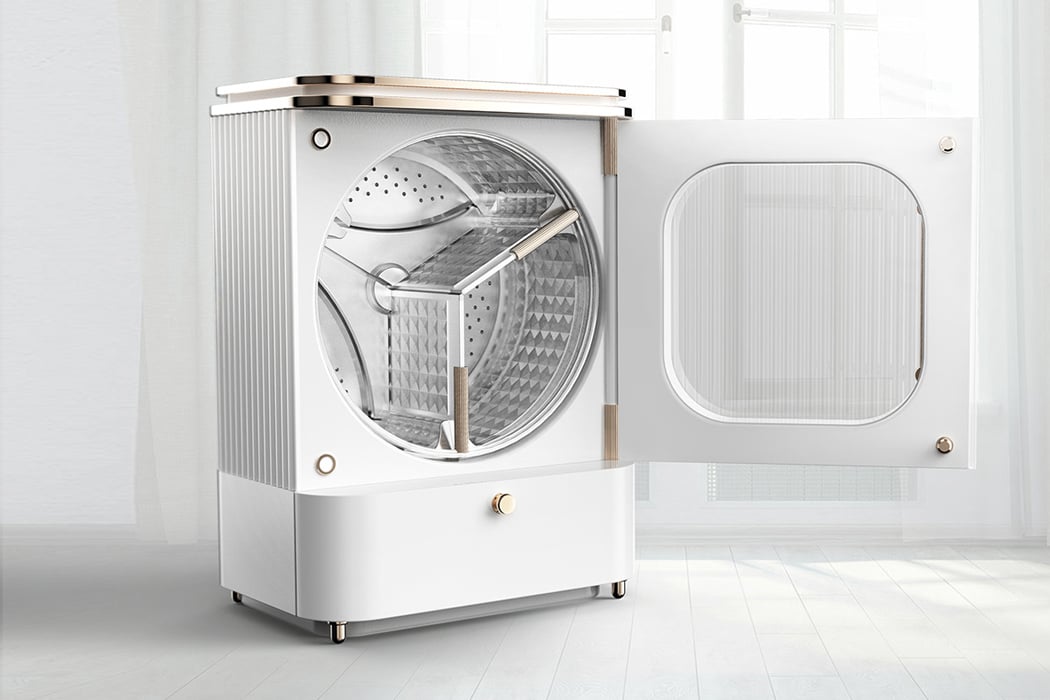The image depicts a sleek, front-loading dryer with a primarily white and silver design. The machine's front features an open door with a clear glass window, offering a view of the polished silver drum interior. Notably, the dryer is topped with a silver panel and supported by small silver legs, with a distinctive gold knob situated near the bottom. The scene is set against a pristine white background, with a white floor and a nearby window that allows sunlight to cast gentle shadows, adding depth to the image. This clean and modern setup, complete with white curtains framing the window, suggests the photo might be intended for a commercial advertisement. The overall color palette includes whites, silvers, and subtle grays from the ambient light and shadows.